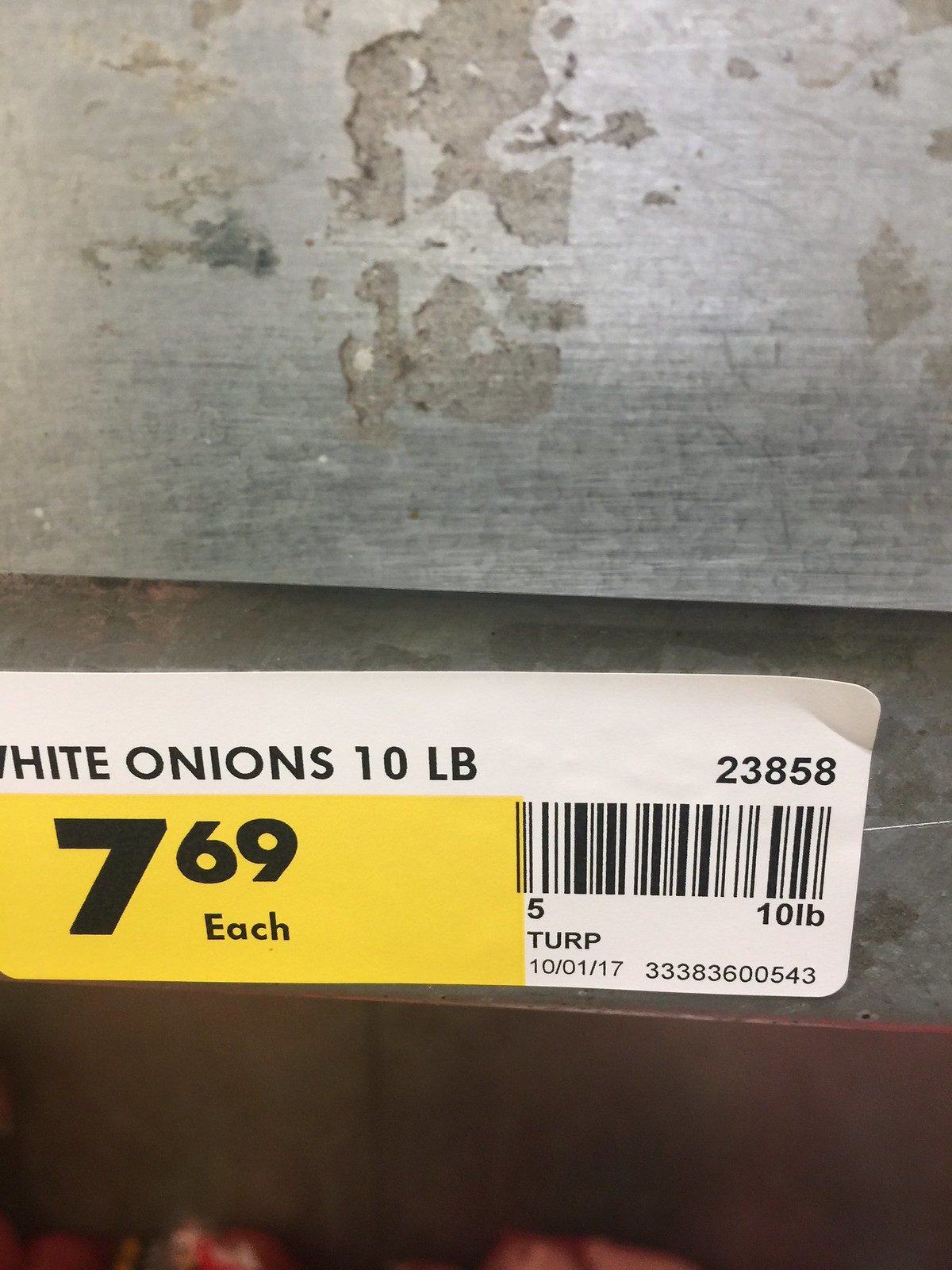This detailed close-up photo captures a retail price tag from a shelf or bin designated for 10-pound sacks of white onions priced at $7.69 each. The tag prominently features large black lettering on a yellow background, indicating "$7.69 each," positioned on the lower left corner. To the right of this pricing detail is a barcode, accompanied by the item number "333-836-00543." Above the barcode, additional text displays "TURP 10-1-17," which is likely a date. The upper portion of the sticker is white, with "White Onions, 10 pound" and the number "23858" clearly printed in black. Despite the visible, slightly worn wooden or possibly steel edge of the shelf or bin, the image does not show any onions, emphasizing the designated storage area for the produce. The tag is affixed to the divider, aiding in the organization and identification within the retail setting.